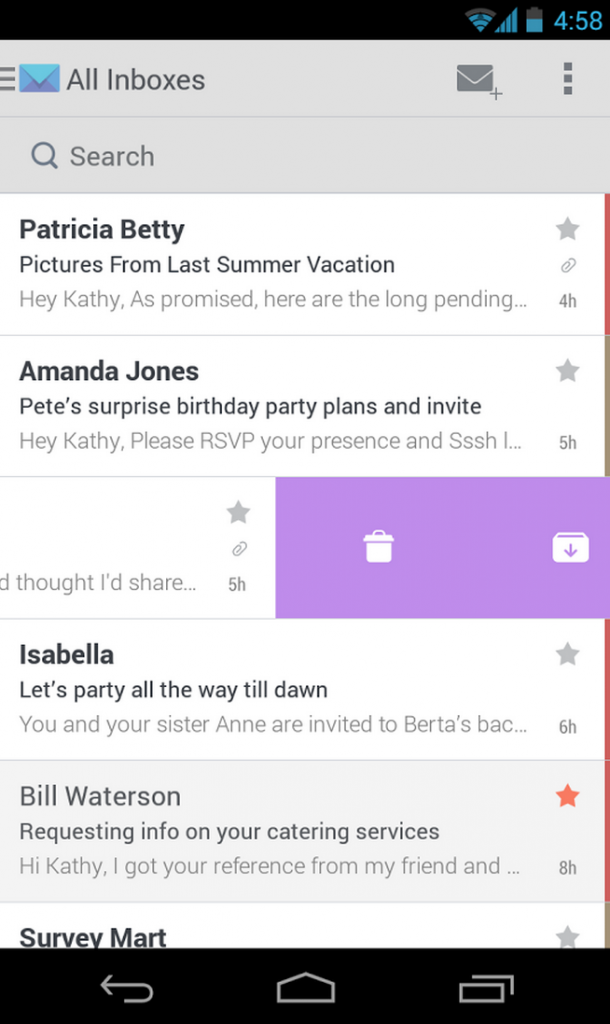This image is a screenshot of an email application on a cell phone. The screenshot is vertically oriented, with its height exceeding its width. The screen capture shows only the digital display, without any part of the physical phone being visible.

At the top of the image, there is a thin black bar displaying essential phone indicators in blue: signal strength, cellular data status, battery level, and the current time, which is 4:58. Below this, there is a slightly larger black bar at the bottom, possibly indicating the phone’s navigation controls.

Directly below the top bar, a gray area contains two rectangular boxes. The first box features a blue envelope icon followed by the text "All inboxes" in gray. To the right of this text, there is another gray envelope icon and a set of three vertical dots, likely representing more options. Directly beneath this, there is a "Search" bar for filtering through emails.

The main section of the screen displays a list of emails:
1. The first email is from Patricia Betty with the subject "Pictures from last summer vacation." The preview snippet reads, "Hey Kathy, as promised here, the long pending..." Additionally, there is a paperclip icon, indicating an attachment, and a timestamp showing the email was received 4 hours ago. 
2. Following this, there is an email from Amanda Jones.
3. The third email is notably half slid to the left, exposing a purple background on the right side, suggesting that the user might be archiving or deleting it.
4. Other visible emails are from Isabella, Bill Waterson (already read and starred), and Survey Mart.

This detailed snapshot offers insight into the email application's interface and the user's recent correspondences.